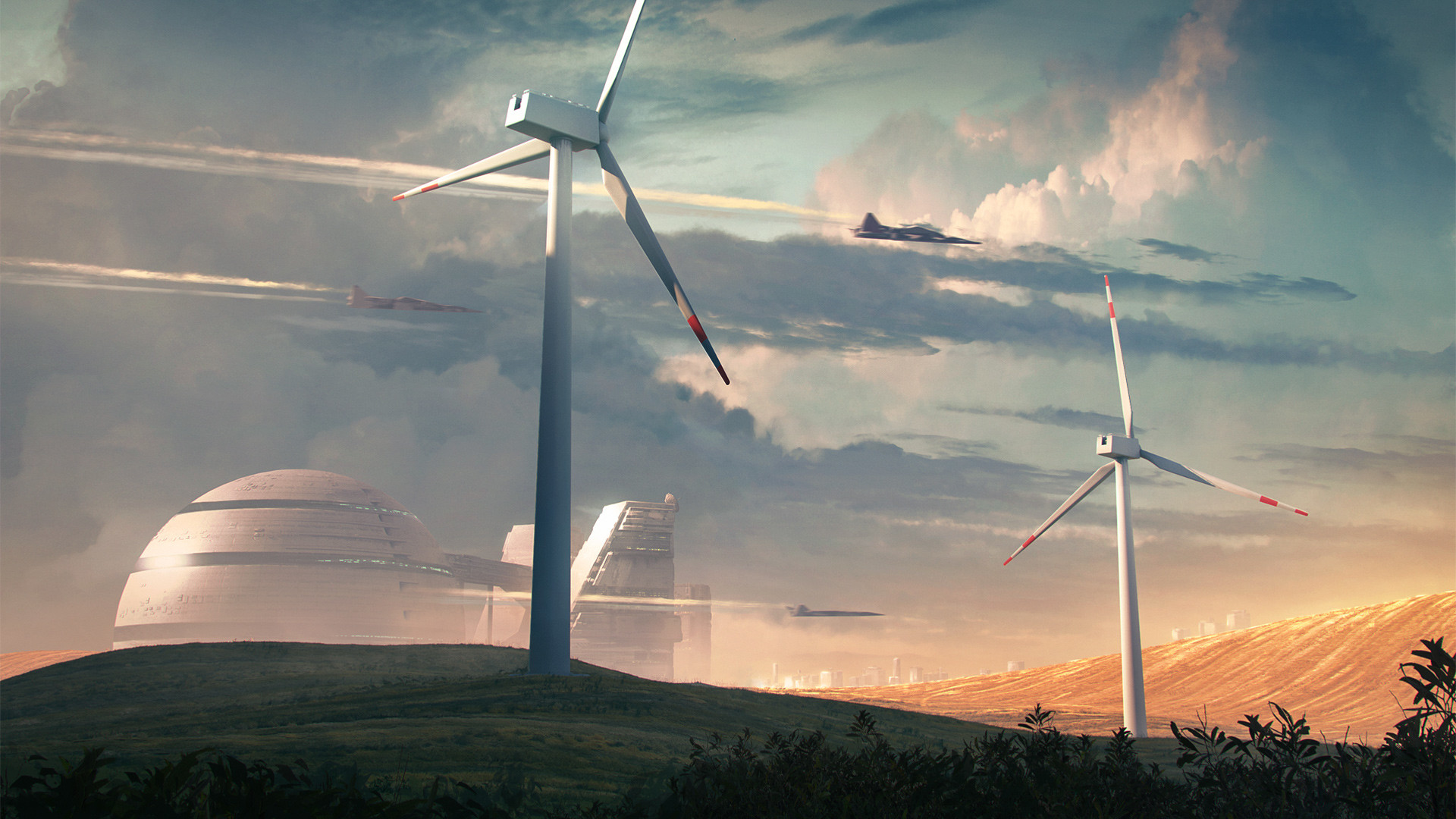The image is a highly detailed, futuristic digital painting or illustration set in an arid, almost desert-like landscape. In the foreground, there are two large wind turbines with red-tipped, three-bladed propellers. The first turbine is prominently situated toward the center left, stretching almost the full height of the image, with one blade extending out of the frame. The second turbine is positioned farther back and appears smaller due to its distance.

Behind these wind turbines, a rolling hill rises, dominated by an imposing structure that features a large, spherical dome reminiscent of the Death Star from Star Wars. The dome is white to gray and is flanked by additional geometric, polygonal structures on the right. 

Cutting dramatically across the scene are three fighter jets, casting vapor trails as they streak by at high speed. One jet flies particularly low to the ground, enhancing the dynamic atmosphere of the image.

In the background, the sky is filled with many dense, dark clouds interspersed with patches of teal and light blue, adding depth and further emphasizing the fantastical and sci-fi nature of the scene. Small trees in the dark foreground contextually indicate the grand scale of the overall illustration.